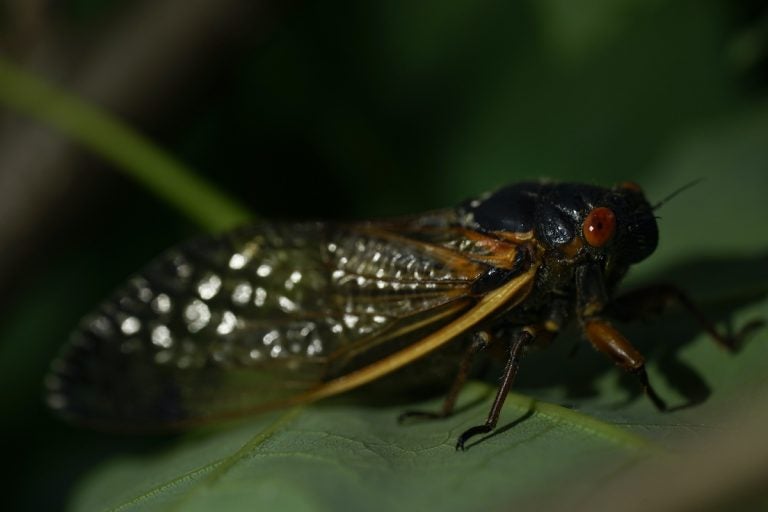This is a close-up photograph of a cicada perched on a slightly blurry green leaf. The image focuses on the insect, highlighting its distinctive features against a dimly lit background. The cicada is oriented to the right, showcasing its bulbous red-orange eyes with small black centers. Its head is pitch black, seamlessly blending into its predominantly black body. The legs extend outward, appearing dark brown to black with subtle hues of dark red. The cicada's large wings, primarily translucent with light brown tops, sprout from behind its head and lie flat against its body, reflecting light and revealing a bumpy texture. The shadow of the insect is visible to the left, adding depth to the image.